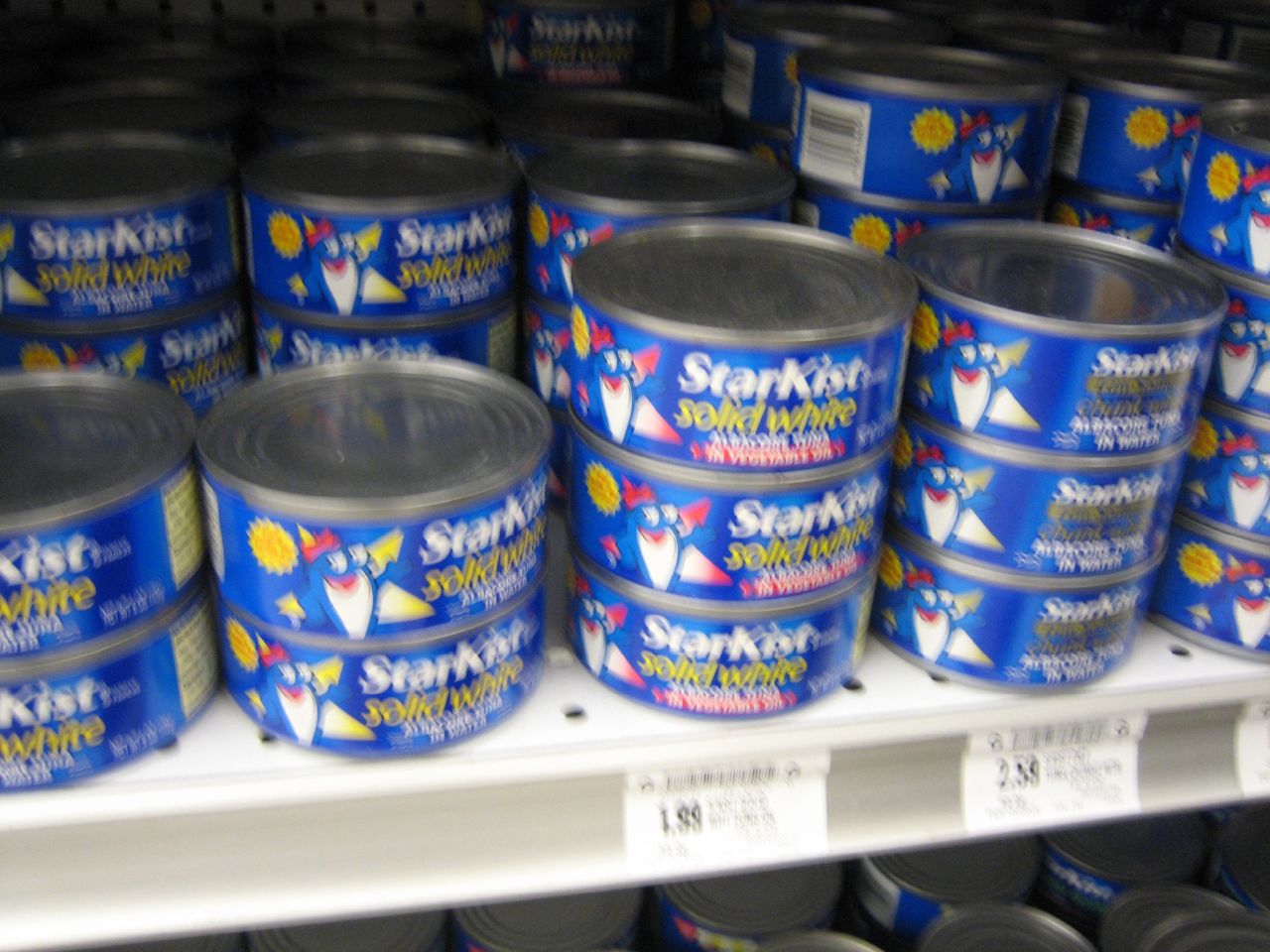This photograph captures a section of a grocery store shelf filled with cans of Starkist solid white tuna. The cans, featuring blue, yellow, and red colors with a cheerful fish mascot, are stacked in varying heights from two to four cans per stack. The white metal shelf has a perforated base with small holes visible throughout. Two white price labels are affixed to the shelf, though the prices are indiscernible due to the overall blurriness of the image. The lower part of the image frames additional cans beneath the shelf, shrouded in darkness and cut off from full view. The upper left corner of the photograph also transitions into shadow as it recedes into the depths of the shelving unit. Overall, the image is out of focus, making finer details hard to discern.